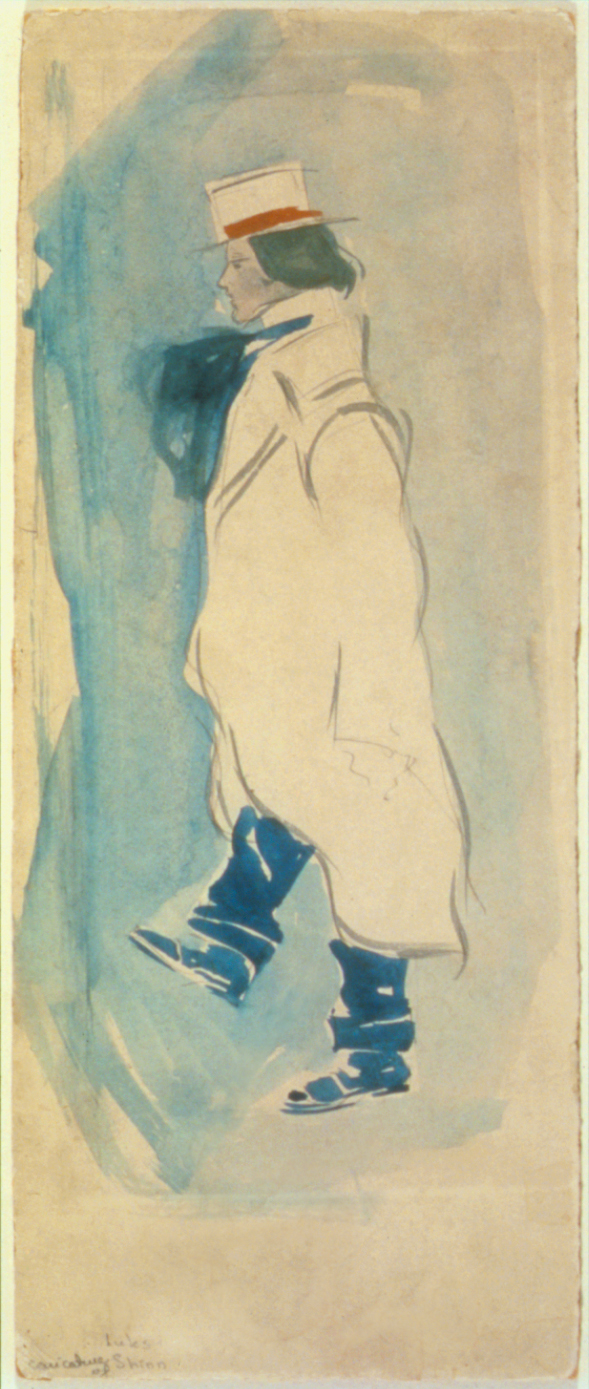The image depicts an abstract, tall and skinny watercolor sketch of a person walking to the left. The figure has traits that suggest ambiguity in gender, but key details align towards a depiction of a man. The individual is wearing a puffy white jacket and a white boxy top hat adorned with a red strap. His face is minimally detailed with a gray color, small black dots for eyes, and thin lines for eyebrows, with only part of his nose visible. His gray hair peeks out from under the hat. A dark blue smudge resembling a bow tie is visible at the neck. 

One of his legs is raised, while the other remains on the ground, colored with blue marker, suggestive of boots. The background is a mix of light blue and off-white colors. At the bottom left corner, a faded brown cursive signature is present, although illegible. The overall aesthetic blends the simplicity of pencil sketching, bolder marker lines, and the fluidity of watercolor, rendering a nostalgic, possibly 1920s-inspired impressionist feel.